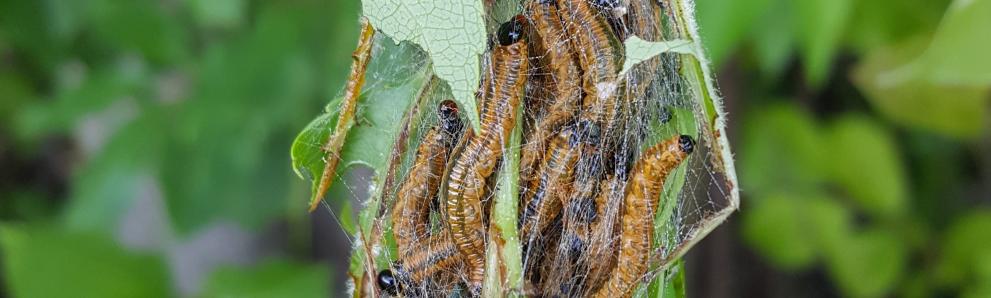This detailed close-up photograph captures a cluster of caterpillars, likely future butterflies or moths, enclosed within a transparent, web-like cocoon hanging off a tree branch. The web appears as a protective net, interwoven with tree leaves, providing a critical habitat as the caterpillars progress from larvae to their next stage of metamorphosis. The caterpillars, each sporting a dark black head and a long, slender brown body accented by two dark brown stripes with a lighter middle stripe, number around eight to nine. The background, though blurred, reveals a lush green setting suggestive of a woodland environment. For now, these caterpillars will continue to feed voraciously on the surrounding tree leaves, contributing to the life cycle before they eventually transform and take flight.